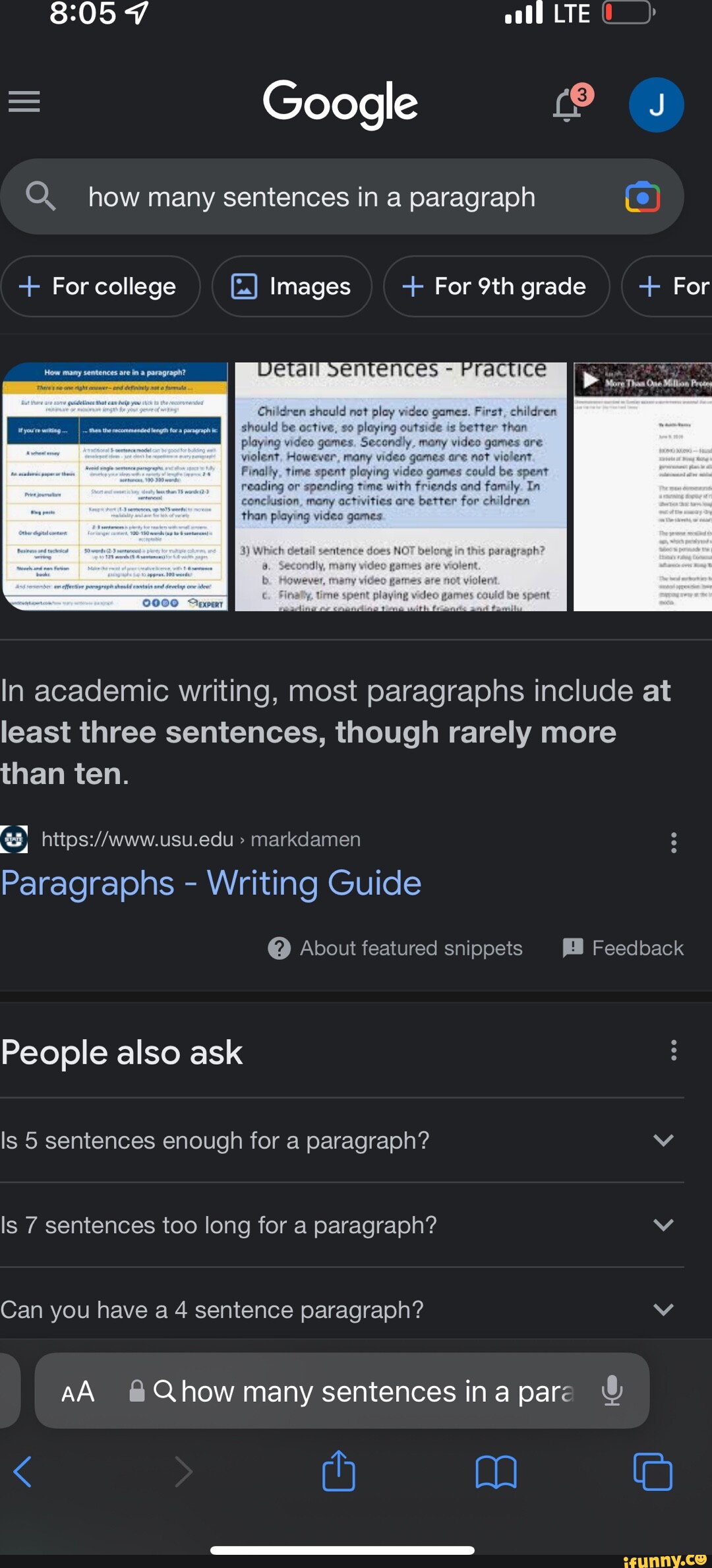This is a detailed screenshot of a mobile device displaying the main Google search page with a dark theme. At the top, the time is displayed as '8:05' in white, accompanied by a location arrow. To the right, four bars signify signal strength next to an LTE indicator, and an almost empty battery icon shows a hint of red, indicating low battery.

Below this status bar, the interface features a Google search bar. On the left of this bar are three horizontal lines in gray, representing the menu. In the center, 'Google' is prominently displayed in white. On the right, there is a bell icon with a red notification badge showing the number 3, followed by a blue circle with a white 'J' inside, denoting the user's profile. 

Within the search bar itself, which is a lighter gray, there is a gray magnifying glass icon followed by the search query text "how many sentences in a paragraph". Next to this, there is a camera icon and three full speech bubbles containing a mix of images, including four college-related and four ninth-grade related pictures.

Immediately below the search bar, Google presents three images as part of its search results. Underneath these images, there is a piece of featured text in gray: "In academic writing, most paragraphs include at least three sentences, though rarely more than ten." This is followed by a blue link titled "Paragraphs - Writing Guide" along with other blue text options for "about featured snippets" and "feedback."

Further down the page, there is a "People also ask" section, featuring three expandable drop-down menus with the questions: "Is five sentences enough for a paragraph?", "Is seven sentences too long for a paragraph?", and "Can you have a four-sentence paragraph?"

The screenshot cuts off at the main search bar at the bottom, which includes text partially reading "how many sentences in a para," followed by a microphone icon. Below this search bar, there are five icons: a blue left arrow, a gray right arrow, a blue share icon, a blue bookmark icon, and two overlapping blue squares for managing multiple tabs. A white bar at the bottom indicates where you can swipe up for additional options or the app drawer.